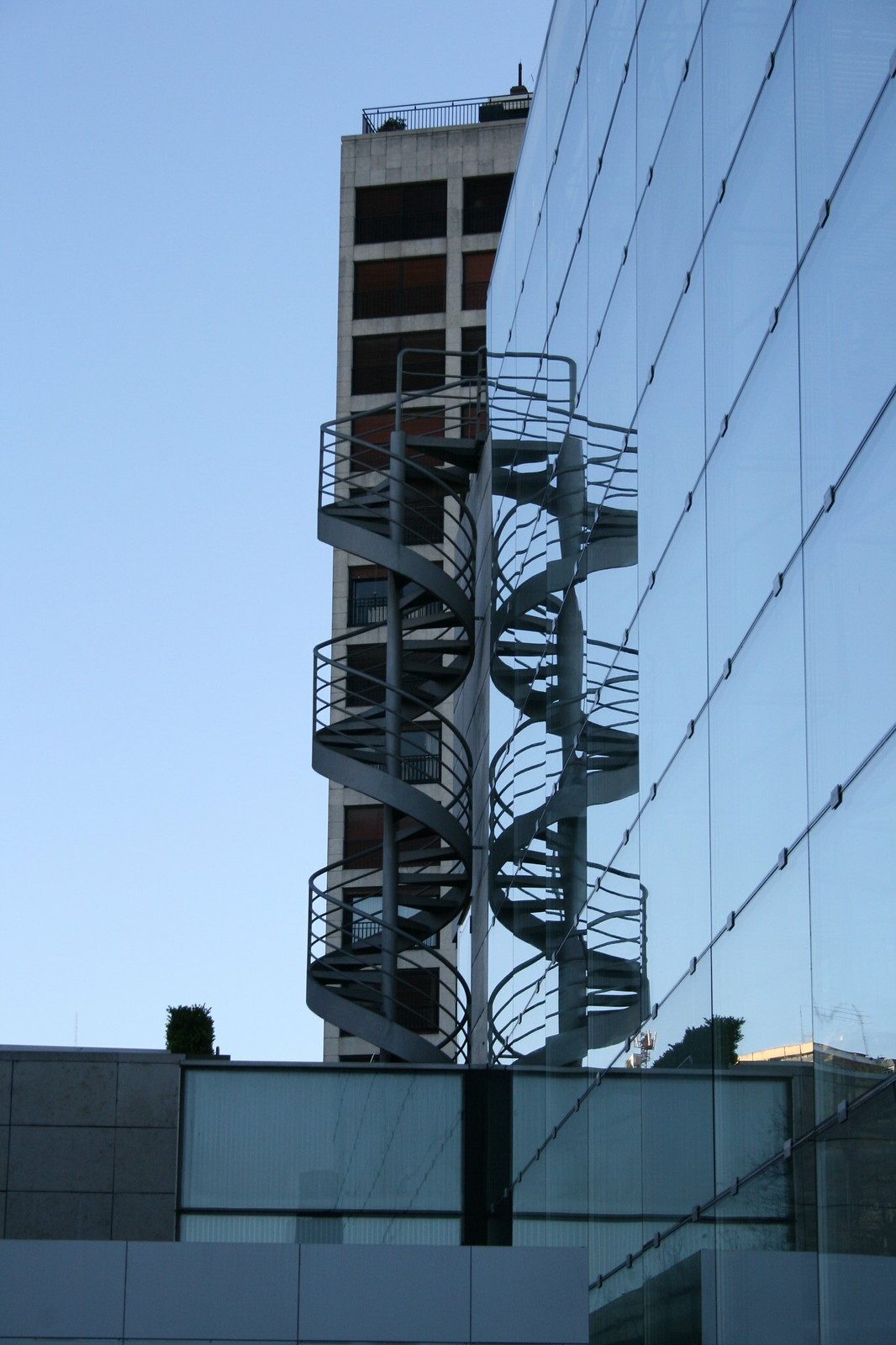The photograph captures a modern, elegant city building in a downtown area with reflective glass windows covering the entirety of its right-hand side. Dominating the center of the image is a striking metal spiral staircase, which climbs almost the entire length of the building and features handrails with a sleek, ribbon-like design. The staircase, both essential for utility and visually captivating, is cleverly mirrored in the glass exterior of the building. Adjacent to this, a smaller cube-like section of the same building, featuring square geometric shapes, incorporates other materials like concrete or metal. The clear blue sky, devoid of any clouds, highlights the stark yet sophisticated aesthetic of the structure. In the background, a taller skyscraper with large black windows can be seen, its height towering over the reflective glass building. Also visible is another building, likely a parking garage with cutouts and a fence on top, adding to the layered urban landscape.